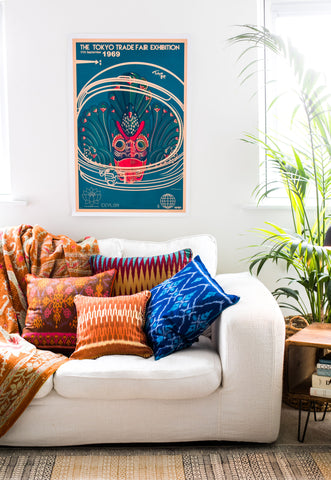This photograph captures a vibrant and stylish living room, dominated by a plush, low-backed white fabric couch adorned with four distinctive decorative pillows. The pillows feature bold designs: a bright blue pillow with intricate blue patterns, an orange pillow with white and orange motifs, a red pillow with pink and orange accents, and a partially hidden pillow exhibiting blue, red, and orange zigzags. To the left of the couch drapes an orange blanket embellished with yellow, red, and orange designs. Centered above the couch on the white wall hangs a framed poster from the Tokyo Trade Fair Exhibition 1969, showcasing a whimsical pink owl with a pineapple on its head, set against a teal background. Flanking either side of the central artwork are windows framed by white trim. To the right of the couch sits a small wooden coffee table with black iron legs, partially visible with books placed on it. Adjacent to the table stands a lush houseplant with tall green leaves. The floor features a beige and dark-colored rug with a dynamic pattern, enhancing the room's overall aesthetic.